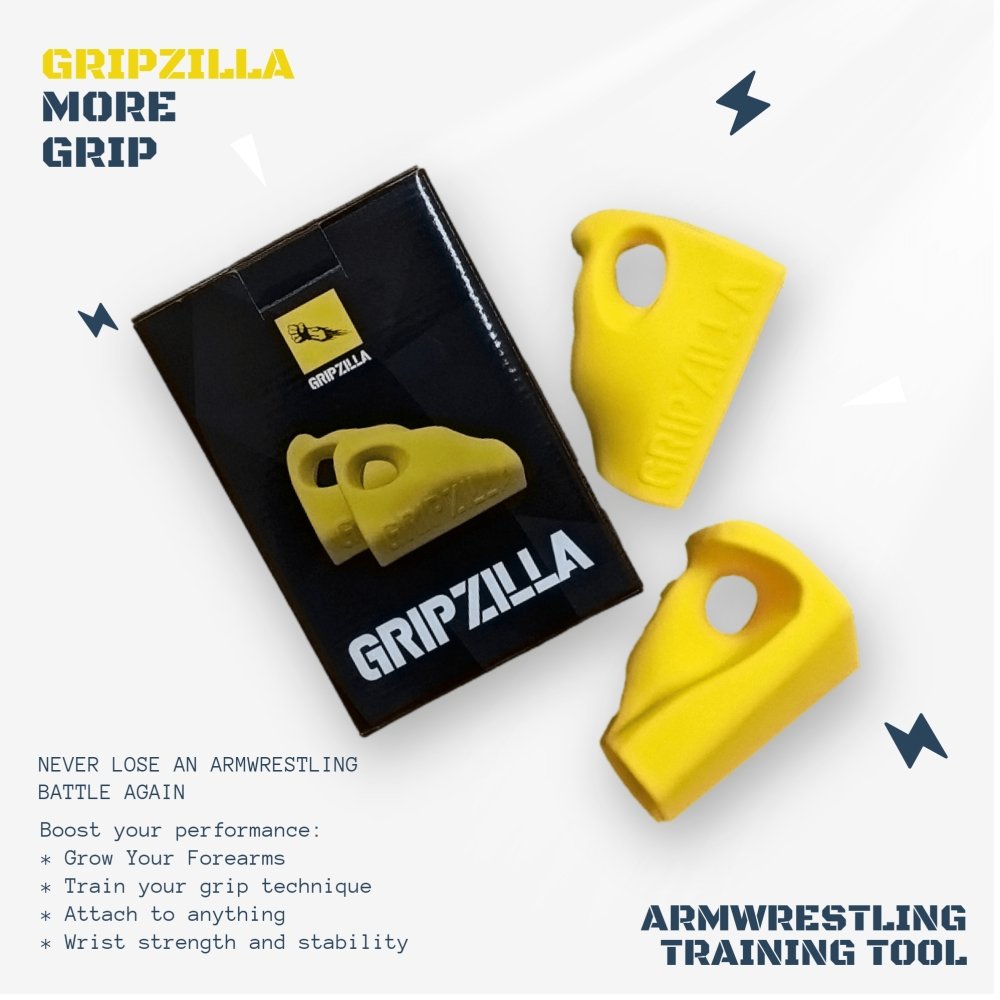The advertisement for Gripzilla prominently features a sleek black box adorned with the Gripzilla logo, showcasing two striking yellow Gripzilla arm wrestling training tools. These tools, molded to fit the hand with thumb access ports, promise enhanced grip strength and wrist stability. The box's top left corner highlights the product name 'Gripzilla' in bold yellow, followed by the tagline 'More Grip' in black. Lightning bolts in blue add a dynamic touch, emphasizing the product’s power. The bottom left corner features motivating phrases in stencil font: "Never lose an arm wrestling battle again. Boost your performance. Grow your forearms. Train your grip technique. Attach to anything," underlining Gripzilla's multifunctional benefits.